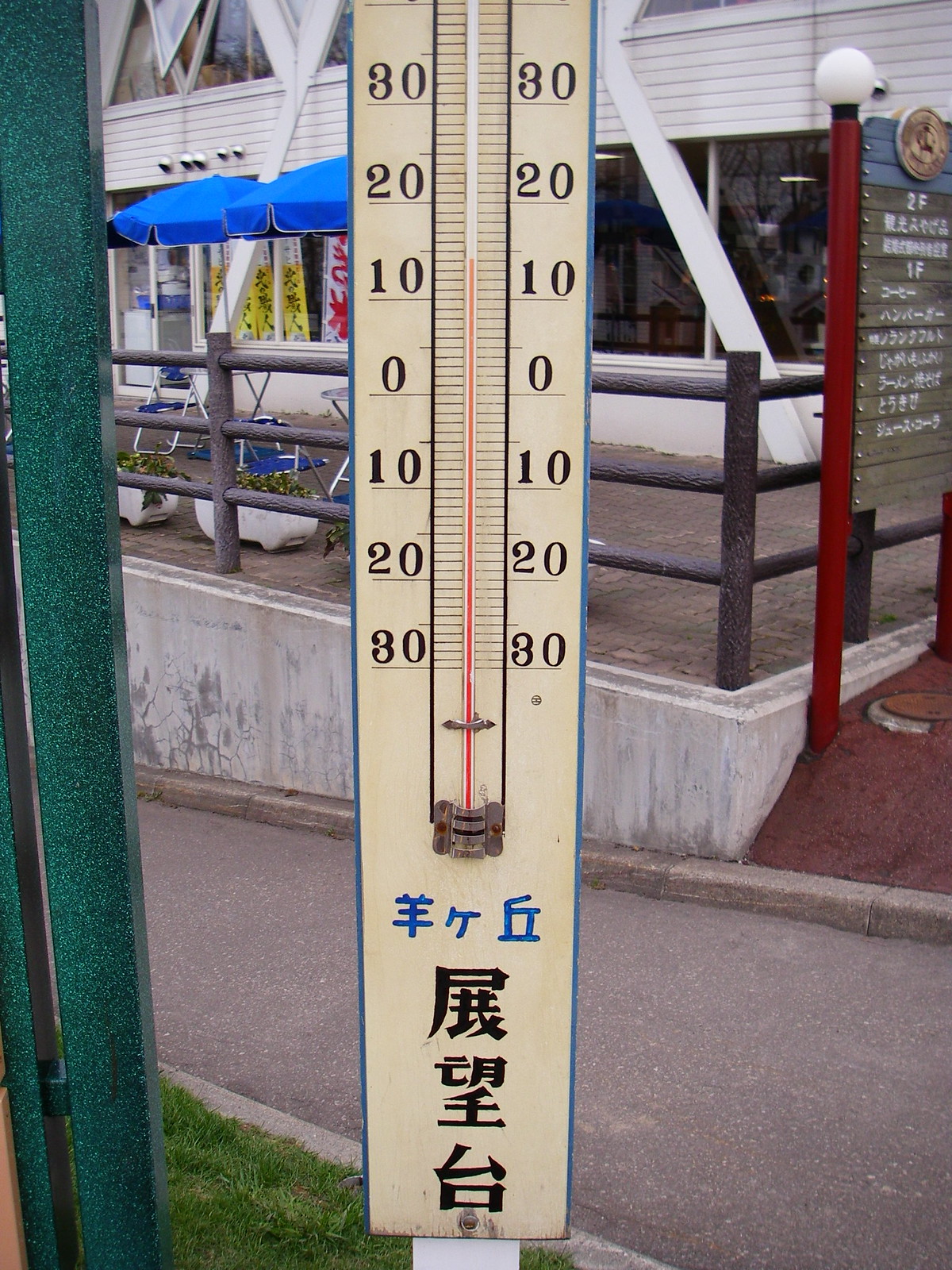The image depicts a large outdoor thermometer, which appears to be situated in China due to the Chinese characters visible at its base. The thermometer uses standard Arabic numerals to display the temperature, which is around 14 degrees Celsius. 

In the background, there is an outdoor seating area that seems to belong to a shop or a small strip of shops. A board listing the names of these shops is noticeable, indicating the presence of a commercial area. There is also a walkway behind the thermometer, approximately four feet wide, leading past the shops. 

The thermometer is positioned on a grassy area and is flanked to the left by a green pole or metal structure. Additionally, one of the buildings in the background houses an observable piece of machinery, contributing to the bustling ambiance of the location.